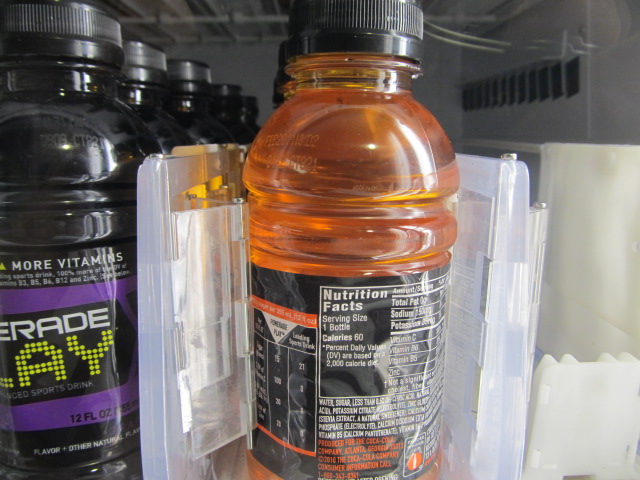The image captures the interior of a refrigerator, potentially within a vending machine. Central to the scene is an orange drink featuring a black cap and a black label displaying nutritional facts. This drink is part of a row of similar orange bottles extending into the background. To the left of the orange drink, there are black bottles with black and purple labels, though part of the logo on these labels is obscured. The right side of the image reveals an empty shelf with no items placed on it.